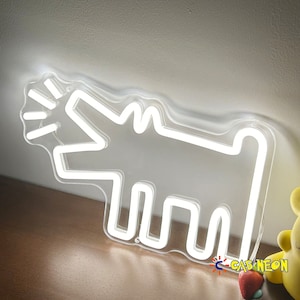This square-format color photograph features a stylized, neon sign shaped like a barking dog. The artwork, primarily white in color, is crafted from a material resembling plastic or resin, rather than traditional glass neon. The dog is depicted in profile with its mouth open, facing the upper left corner of the image. Four straight lines emanate from the mouth to symbolize barking. The dog is characterized by its simple, blocky features, including four legs, two pointy ears, and a tail positioned on the right side of the composition. The neon sign is mounted on a clear plastic background and leans against a white wall, resting on a dark brown laminate surface. To the right of the sign are a strawberry and a teddy bear toy, while the bottom right corner of the image includes the text "C Gas Neon." The overall setting appears to be indoors, suggesting a product photo, possibly for an online marketplace.